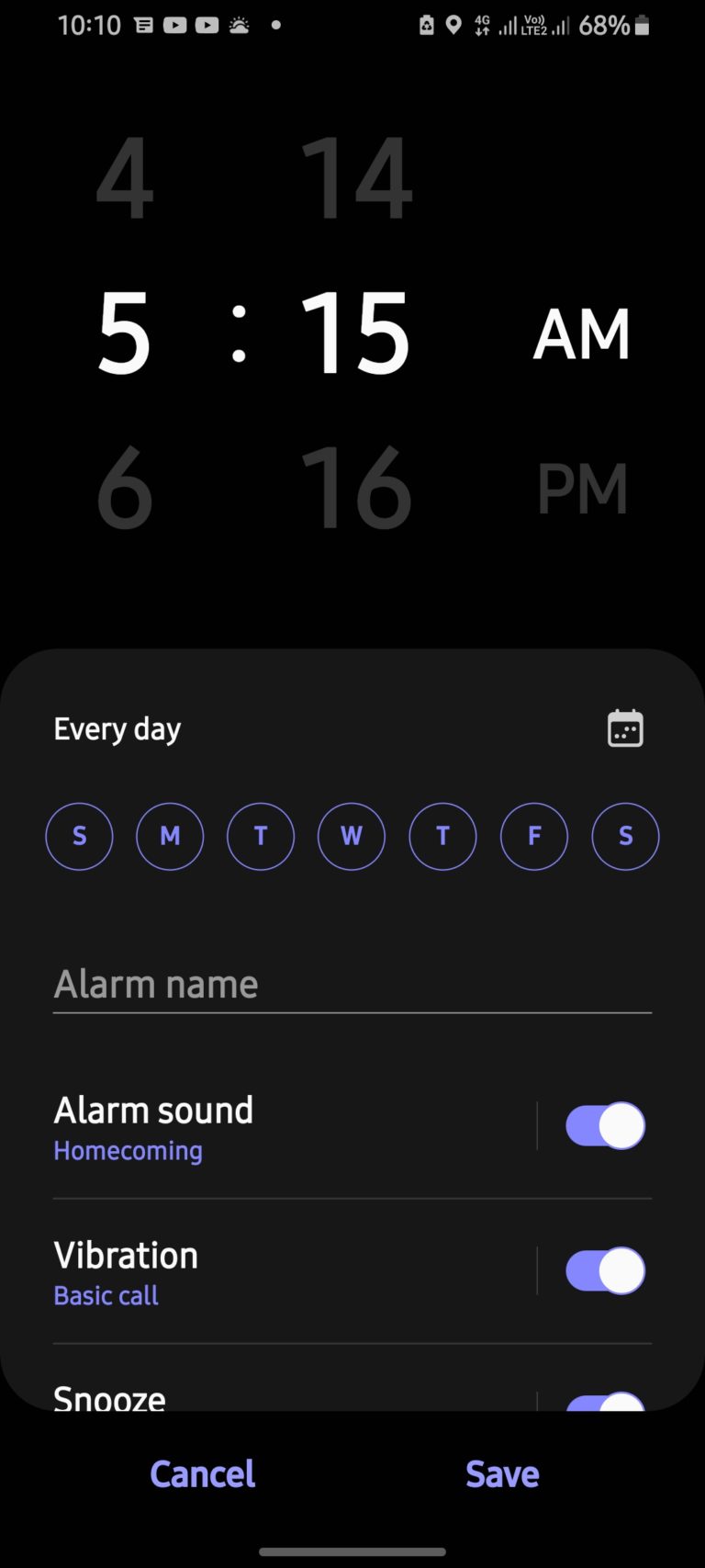A close-up image of a smartphone against a solid black background showcases the device’s alarm setting interface. In the top left corner, the clock reads 10:10, with various system icons—such as a 4G indicator, network strength bars, VoIP connection, Wi-Fi signal, and battery life at 68%—aligned on the right-hand side. Below this, the current time is digitally displayed as 5:15 AM, indicating the selected alarm time.

The screen features a grey panel filled with adjustable options for the alarm. The first option allows users to set the alarm to repeat on specific days, with choices ranging from Sunday to Saturday. The alarm can be personalized with a name and set to play a specific sound, in this case, "Homecoming." Vibration can also be activated, currently set to "Basic Call." Additionally, there is a snooze option for added convenience. At the bottom of the screen, there are two buttons in a striking purple hue: “Cancel” on the left and “Save” on the right, completing the interface.